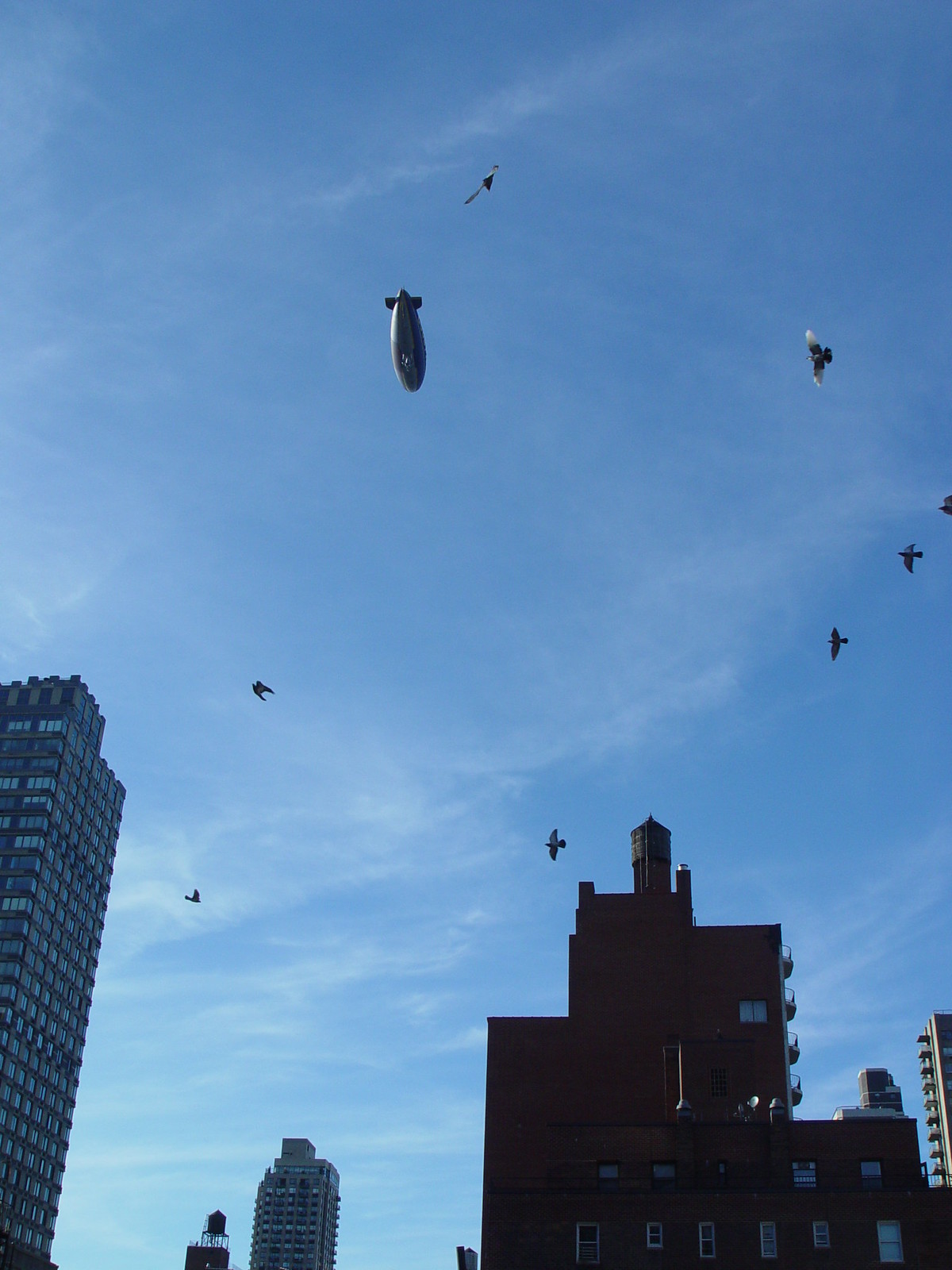The image captures a stunning outdoor scene dominated by a vibrant blue sky softly streaked with wispy white clouds. The skyline at the bottom reveals a metropolitan area, likely New York, as indicated by the presence of cylindrical water towers atop taller residential buildings and condominiums. Skyscrapers, including a vertically tilted one on the lower left, span the bottom edge, with another prominent structure on the lower right, all rendered in varying shades of gray. Birds in flight are scattered across the sky, totaling around ten, with a few forming a V pattern on the right-hand side. Near the top center of the image, a blimp, mistaken by some for an atomic bomb, drifts away, its tail fin and a trailing banner discernible, adding an intriguing focal point to the serene skyscape.